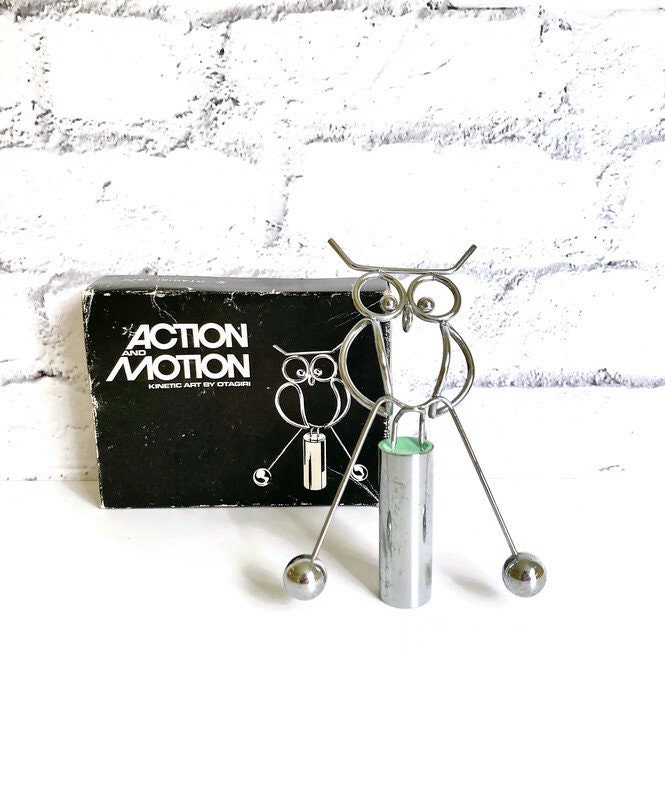The image showcases a kinetic art piece titled "ACTION & MOTION" by Otagen. The main focus is a metal sculpture of an owl with a whimsical, cartoonish design, characterized by long, wire-formed legs ending in circular feet. The owl balances on a cylindrical metal post with two prongs resting on top, implying motion when given a push. This art piece is positioned in front of a slightly worn, black rectangular box, which prominently features the labels "ACTION & MOTION" in all caps and "KINETIC ART by Otagen" in white font. The background consists of a heavily overexposed, white-painted brick wall, which contrasts with the darker, sharper details of the box and the sculpture, making the art piece the primary visual focus.